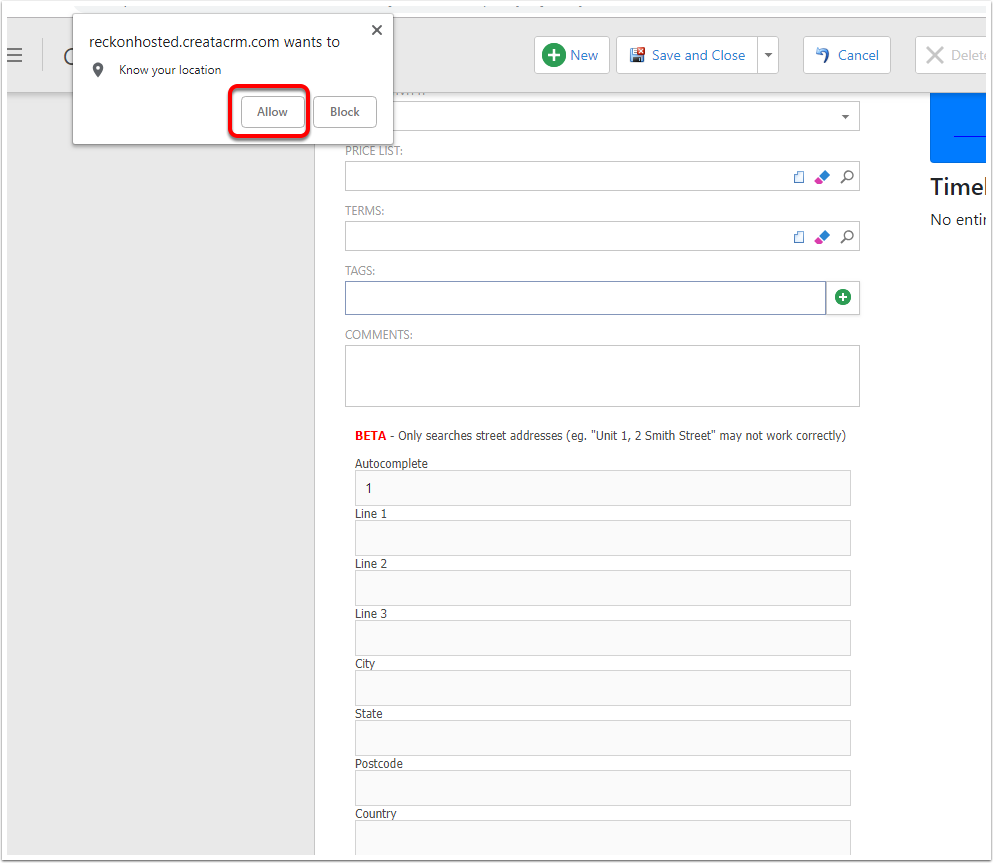Below is a detailed and cleaned-up caption for the image described:

---

The image displays a webpage obstructed by a pop-up notification from reconhosted.credocrm.com requesting permission to access the user's location. The pop-up features a map pin icon accompanied by text reading "know your location" and presents two options: an "Allow" button and a "Block" button, both in gray. A red rectangle highlights the "Allow" button, indicating the user's required action to proceed.

Above this pop-up, several interface buttons are visible in a gray toolbar. From left to right:
- A "New" button, depicted as a circle with a white plus sign.
- A "Save and Close" button represented by a disk icon with a red circle and white X, which includes a dropdown menu for additional options.
- A blue "Cancel" button with a leftward-turning arrow.
- A "Delete" button, currently grayed out and inactive.

Below are multiple input fields for user information:
- "Pricelist" and "Terms" fields, each featuring three icons: a paper with a folded corner, a highlighter, and a magnifying glass.
- A "Tags" field with a green circle containing a white plus sign.
- A "Comments" box for free text input.

Under these fields, in bold red text, is "BETA," indicating an experimental feature. The text states: "ONLY SEARCHES STREET ADDRESS, example, Unit 1 to Smith Street may not work correctly," followed by the label "Autocomplete" and several aligned text fields for address information, including "Line 1," "Line 2," "Line 3," "City," "State," "Postcode," and "Country."

To the far right, a vertical column displays blue bars and the partially visible title "Timeline." Below this, a truncated word starting with "No ENTRI" is cut off and unreadable.